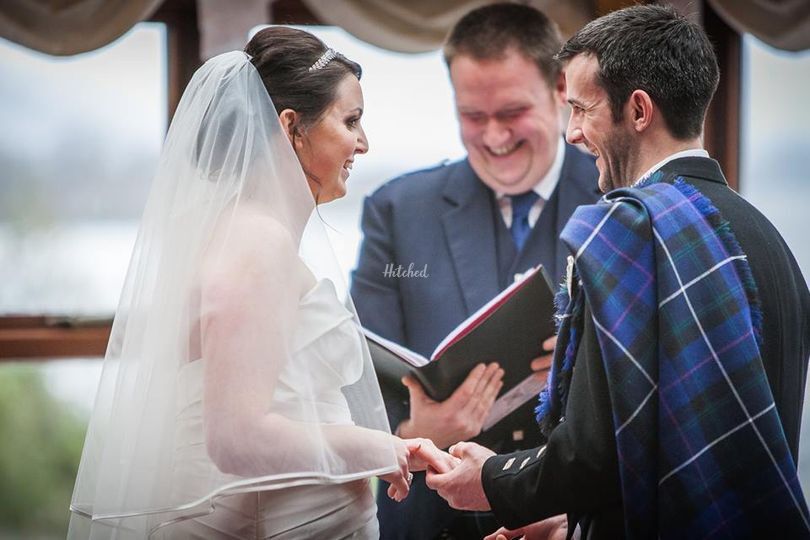The image captures a joyous moment during a wedding ceremony held indoors, illuminated by natural light streaming through a wood-framed window with light brown curtains. To the left stands the bride, a woman with her hair up, adorned with a white veil cascading down the back of her head. She is radiant in a white wedding dress and smiling as she holds the hand of her groom. The groom, positioned to the right, is attired in a black suit, complemented by a colorful tartan sash draped over his left shoulder, featuring a pattern of white, blue, black, green, and purple hues. He looks at the bride with a joyful expression while laughing. In the background, the officiant, dressed in a navy suit with a white-collar shirt and a blue tie, stands smiling and holding a black book, possibly reading the vows. The scene encapsulates the happiness and love shared among those present, with all three individuals beaming with smiles as the couple exchanges their vows.